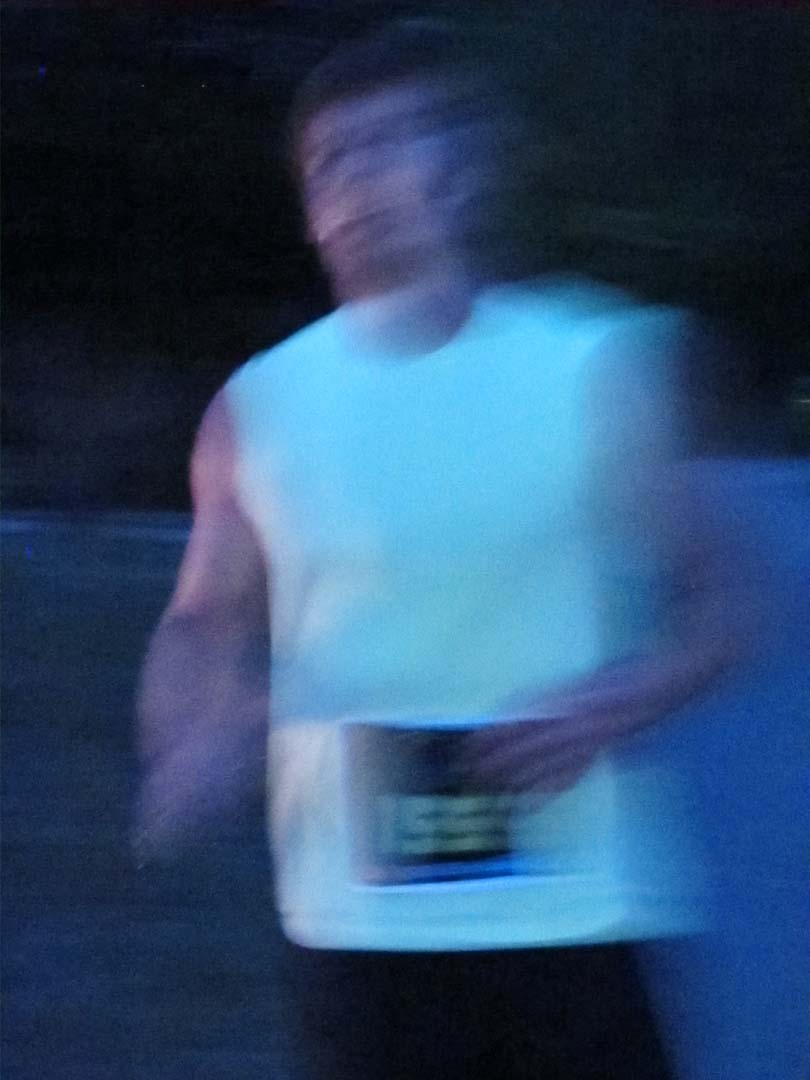A highly blurred photograph captures an indistinct image of a man with dark, possibly curly hair, set against a nighttime backdrop. He exudes a 1950s vibe, mainly due to his attire—a white shirt with sleeves that appear to be rolled up, although it might also be a sleeveless muscle shirt. Notably, there's a rectangular black patch near the bottom of his shirt, displaying the numbers "1, 5, 5" with an obscured final digit and a blue horizontal line beneath it. The man's face and hands are in motion, creating streaks and adding to the overall blur.